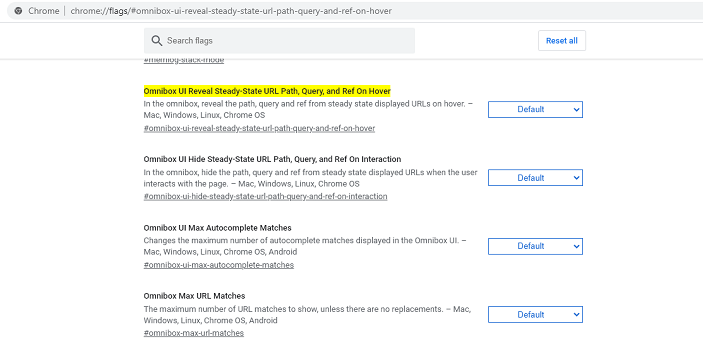A screenshot of the Google Chrome browser interface, specifically the "chrome://flags" page, is displayed. The user is searching for a particular experimental feature flag. The highlighted flag is "omnibox-ui-reveal-steady-state-url-path-query-and-ref-on-hover," which is outlined in yellow in the flag list below. The description provided states: "In the omnibox, reveal the path, query, and ref from steady state displayed URL on hover. Available on Mac, Windows, Linux, and Chrome OS." The setting for this flag is currently set to 'Default'. Additional flags visible in the list include "omnibox-ui-hides-steady-state-url-path-query-and-ref-on-interaction," "omnibox-ui-max-autocomplete-matches," and "omnibox-max-url-matches," all of which are also set to their default settings.